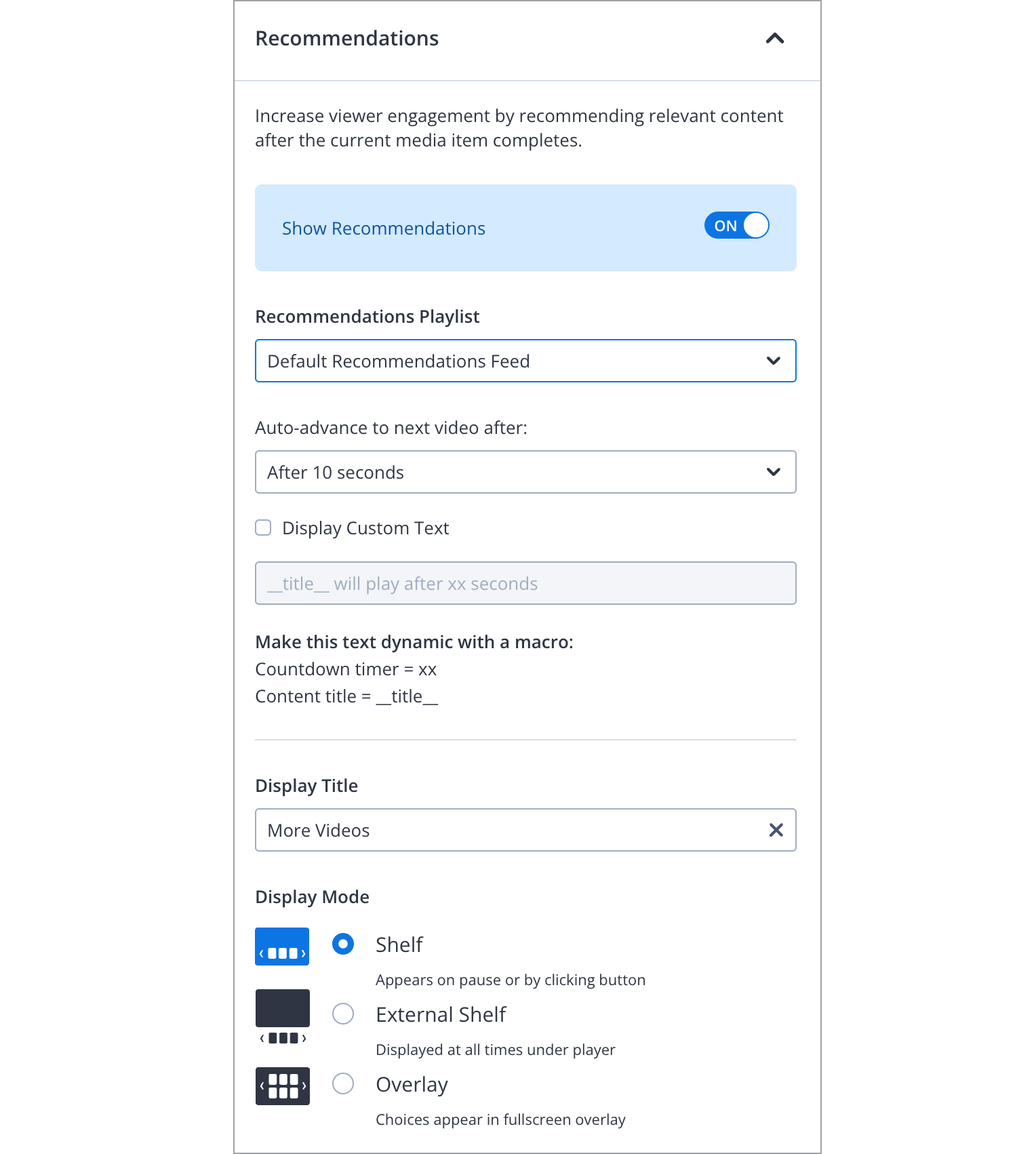The image is a screenshot from a smartphone displaying a recommendation settings page on a media site. The interface is presented on a white, vertically-oriented screen. At the top of the screen, there is a toggle option to either enable or disable recommendations, currently set to "on" and highlighted in a blue pill-shaped bar. 

Underneath the toggle, there is a descriptive prompt stating: "Increase viewer engagement by recommending relevant content after the current media item completes." Directly below this, another blue pill-shaped bar indicates that the recommendation feature is activated.

Next, there's a section labeled "Recommendations Playlist" with a drop-down menu where "Default recommendation speeds" has been chosen. Following this, there's an option titled "Auto advance to next video after," with a selected interval of "10 seconds" from a drop-down menu.

The section "Display custom text" is present but not selected. It also includes an option to "Make this text dynamic with a macro" followed by a description field.

The final category, "Display Title," has "More videos" selected. Additionally, there are three display format options—"Shelf," "External Shelf," and "Overlay," each accompanied by an icon. The "Shelf" option is selected and highlighted in blue.

Overall, the screenshot provides a detailed configuration interface for customizing how media recommendations are displayed to enhance viewer engagement by guiding subsequent content consumption.